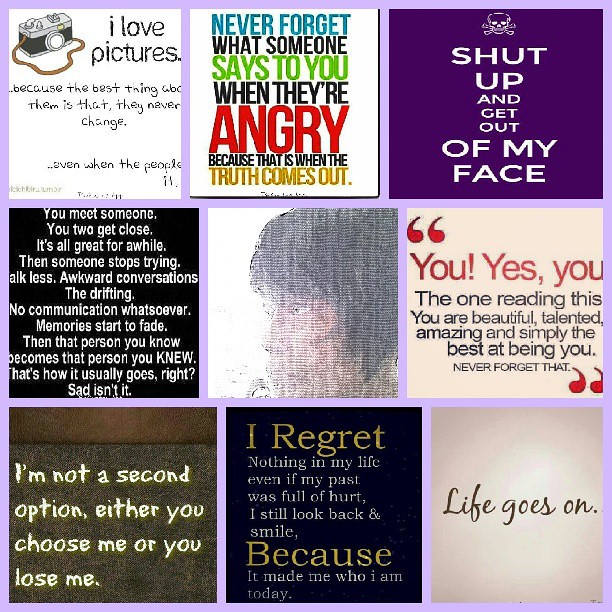This is an image of a 3x3 grid collage, with each square containing a motivational or emotional poster featuring a mix of colors and messages. The overall background is bordered by a purplish-pink color. Here's a detailed description of each square, arranged from left to right, top to bottom:

1. **Top-Left**: This square features an old-fashioned black-and-white camera illustration on a white background, with black handwriting text saying, "I love pictures because the best thing about them is that they never change ... even when the people do."

2. **Top-Center**: A dark purple background with a white skull at the top. Bold white text reads, "Shut up and get out of my face."

3. **Top-Right**: A white background with a striking mix of red, black, green, and orange text. It reads, "Never forget what someone says to you when they are angry, because that is when the truth comes out." Words like "Never forget," "angry," and "truth comes out" are highlighted in blue, red, and orange, respectively.

4. **Middle-Left**: On a black background with white text, it narrates a depressing sequence of events: "You meet someone. You two get close. It's all great for a while. Then someone stops trying. Talk less. Awkward conversations. The drifting. No communication whatsoever. Memories start to fade. And that person you know becomes that person you knew. That's how it usually goes, right? Sad, isn't it?"

5. **Middle**: A faded tan and white background presents the blurred image of a person's face with short black hair. This square doesn't have any textual content clarified.

6. **Middle-Right**: A white square with bold red text at the top saying, "Yes, you! Yes, you!" in quotations. The black text below reads, "The one reading this, you are beautiful, talented, amazing, and simply the best at being you. Never forget that."

7. **Bottom-Left**: This square shows a dark brown leather-like background with white text that states, "I'm not a second option. Either you choose me, or you lose me."

8. **Bottom-Center**: Against a black background, the text is a mix of gold and white: "I regret nothing in my life, even if my past was full of hurt. I still look back and smile because it made me who I am today." Words like "I regret" and "because" are highlighted in bold gold.

9. **Bottom-Right**: A white background with gray script text saying, "Life goes on," accompanied by an illustration associated with the phrase.

Each square uniquely contributes to the overall emotional and motivational theme of the collage, blending textual inspiration with vivid visual diversity.